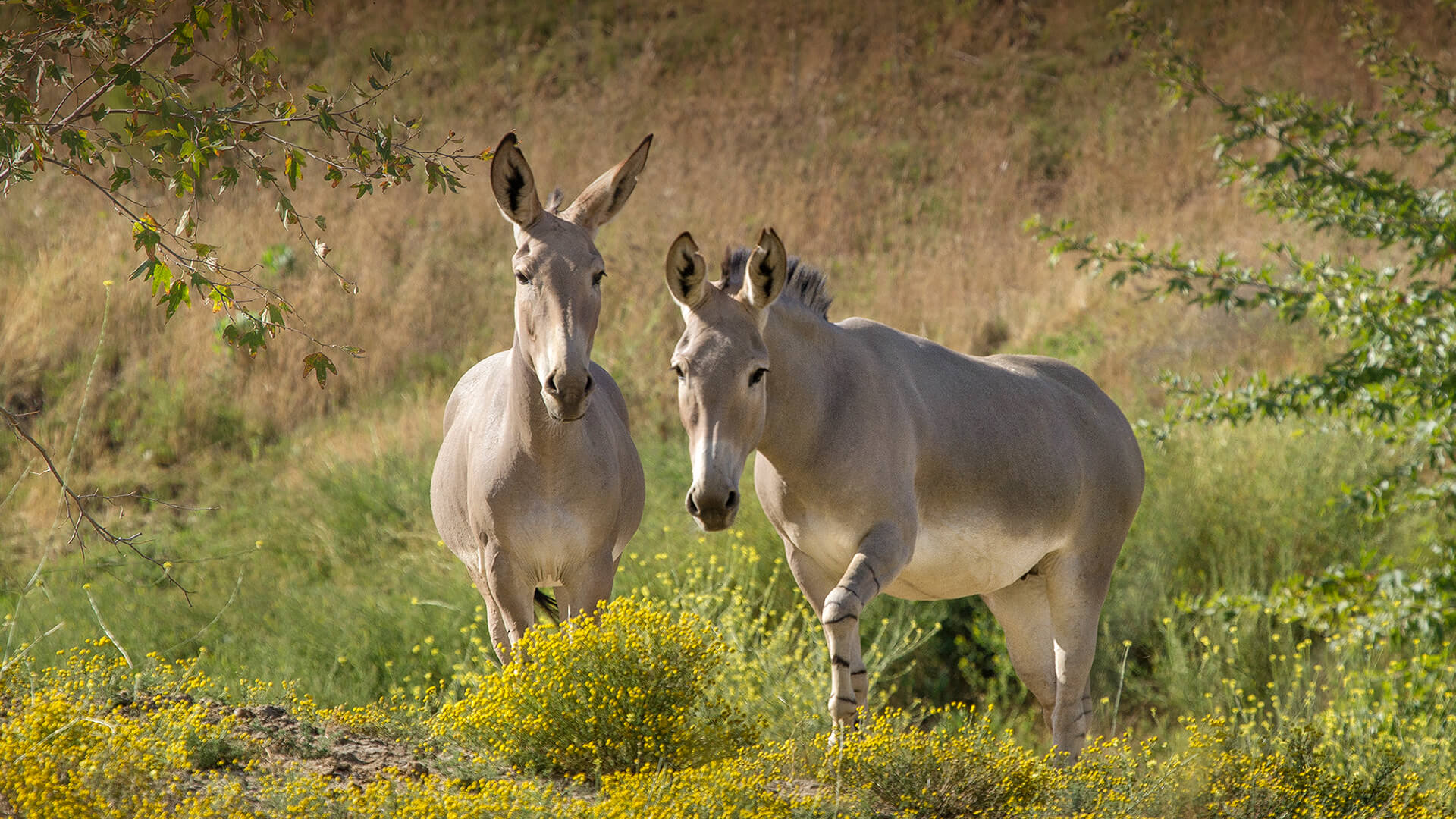In this live photograph, we see two tan-colored donkeys standing closely in a wide, overgrown field dotted with yellow dandelion-like flowers. The donkey on the left, appearing more muscular and well-built, is looking directly into the camera, showcasing its large, upright ears, light khaki fur with some white mixed in, and black lines on its legs. The donkey beside it, positioned diagonally with one of its legs raised, has smaller, rounded ears. The field extends upward towards a larger hill in the background, with patches of green grass and light brown grass interspersed. Tree branches with green leaves frame the scene on both the left and the right, contributing to the natural prairie ambiance of the setting.